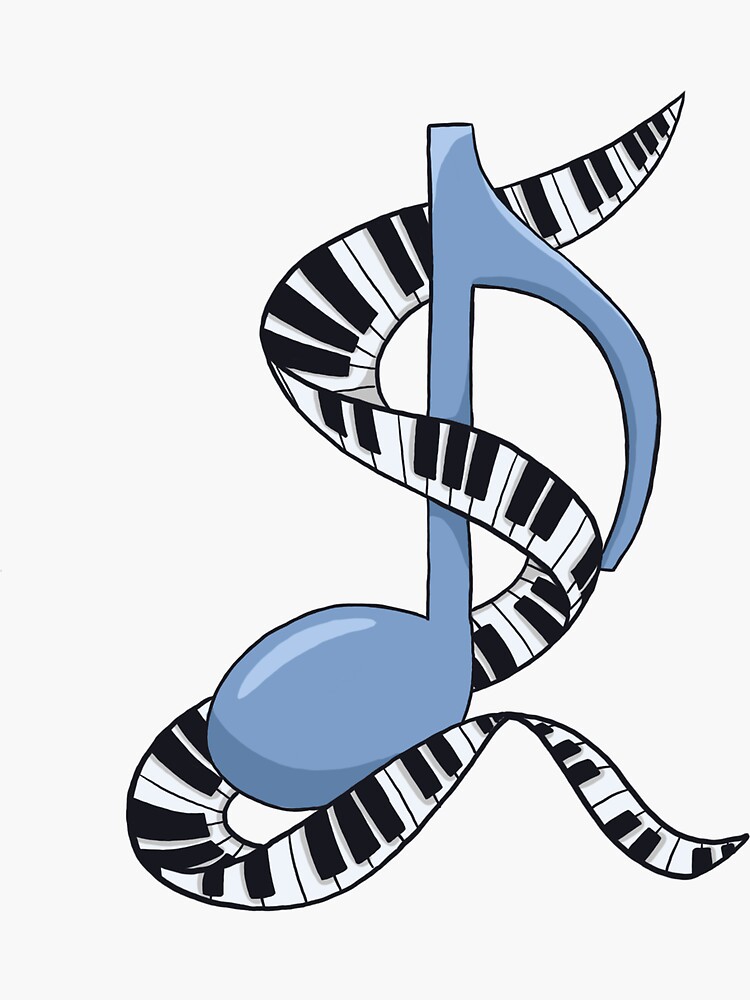This artwork features a large, smoky blue quarter note set against a stark white background. The note is prominently positioned in the center, with its top extending smoothly towards the upper left corner. Ingeniously wrapped around the note is a ribbon-like representation of a piano keyboard, with black and white keys intertwining around the note. This ribbon starts at the upper right, loops behind and above the note, extends underneath it, emerges at the lower left, and then curls back upwards and to the right, evoking the dynamic movement of music itself. The simplicity of the black, white, and blue color palette emphasizes the artistic elegance and musical essence of the piece.